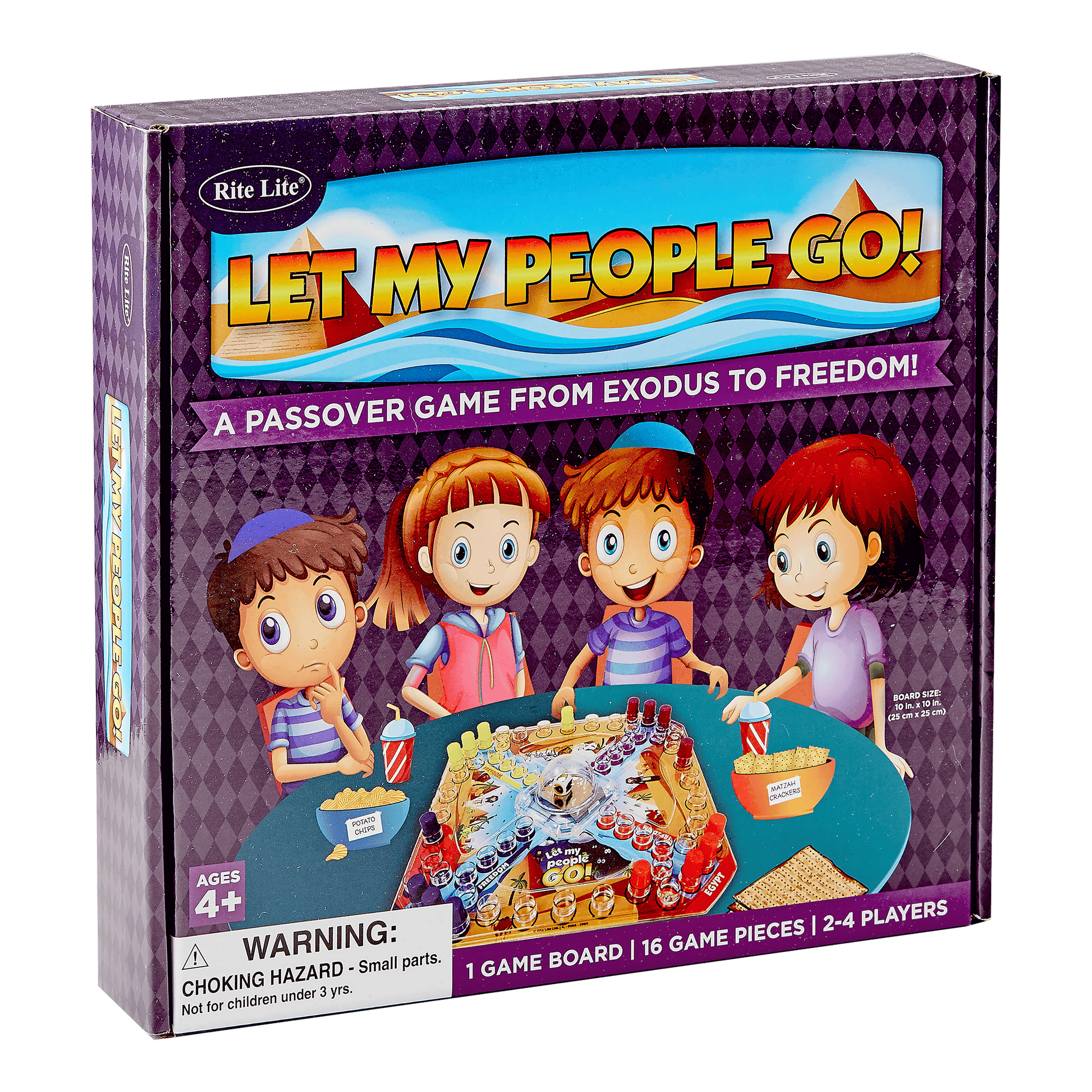This color photograph showcases a board game titled "Let My People Go: A Passover Game from Exodus to Freedom" by Write Life, packaged in a small, CD case-sized box made of cardboard. The box has a striking purple background with the title "Let My People Go" set against a sand and pyramids backdrop in light blue lettering at the top. Beneath the title, in white text, it reads "A Passover Game from Exodus to Freedom," with an illustration of four children below. The children, two boys and two girls, are depicted in a cartoon style, sitting around a round table adorned with snacks like popcorn and drinks. The boys, each sporting blue yarmulkes and striped shirts, sit on the left and second from the right, while the girls have a ponytail and bangs, and shoulder-length hair, respectively. One girl wears a purple shirt while the other has brown hair with a red jumper and blue t-shirt. The game mimics the style of "Sorry," featuring a bubble in the center likely used to roll dice. At the bottom left of the box, there's a white square label with a choking hazard warning about small parts, cautioning against use by children under three years old. Additional details in white text against the purple background specify "Ages 4+, One Game Board, 16 Game Pieces, 2-4 Players."